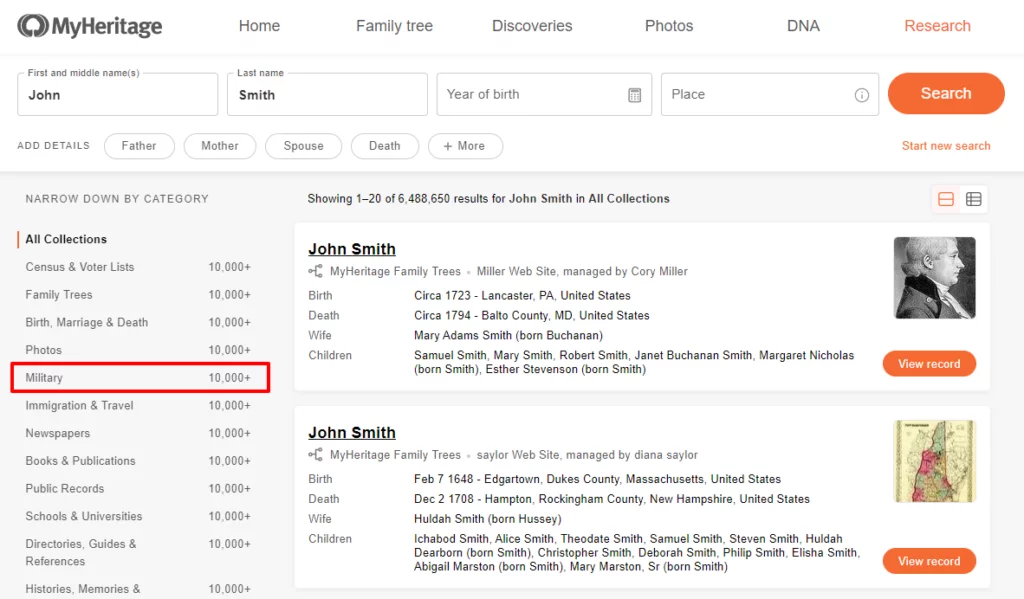The image is a screenshot of a genealogical website interface. In the top left corner is an emblem featuring a white tree encased in a gray circle with the words "My Heritage" to the right of it. To the right side of the screen, there are several navigation options labeled "Home," "Family Tree," "Discoveries," "Photos," "DNA," and an orange-highlighted "Research."

Below this menu, there's a search form with fields for first and middle names, last name, year of birth, and place. The entered information shows "John" in the first name field and "Smith" in the last name field. An orange "Search" button is prominently displayed next to these fields. To the left, there is a section titled "Narrow Down by Category," offering filtering options like "All Collections," "Family Tree," "Birth, Marriage & Death," "Photos," "Military" (outlined in red), "Immigration & Travel," "Newspapers," "Books and Publications," "Public Records," and "Histories, Memories."

In the main part of the screen, the name "John Smith" is underlined, indicating a link. Next to it, there's a black and white side-profile photograph of a president wearing a black collared shirt, with white hair pulled back from his face. Below this photo, an orange button labeled "View Record" is visible.